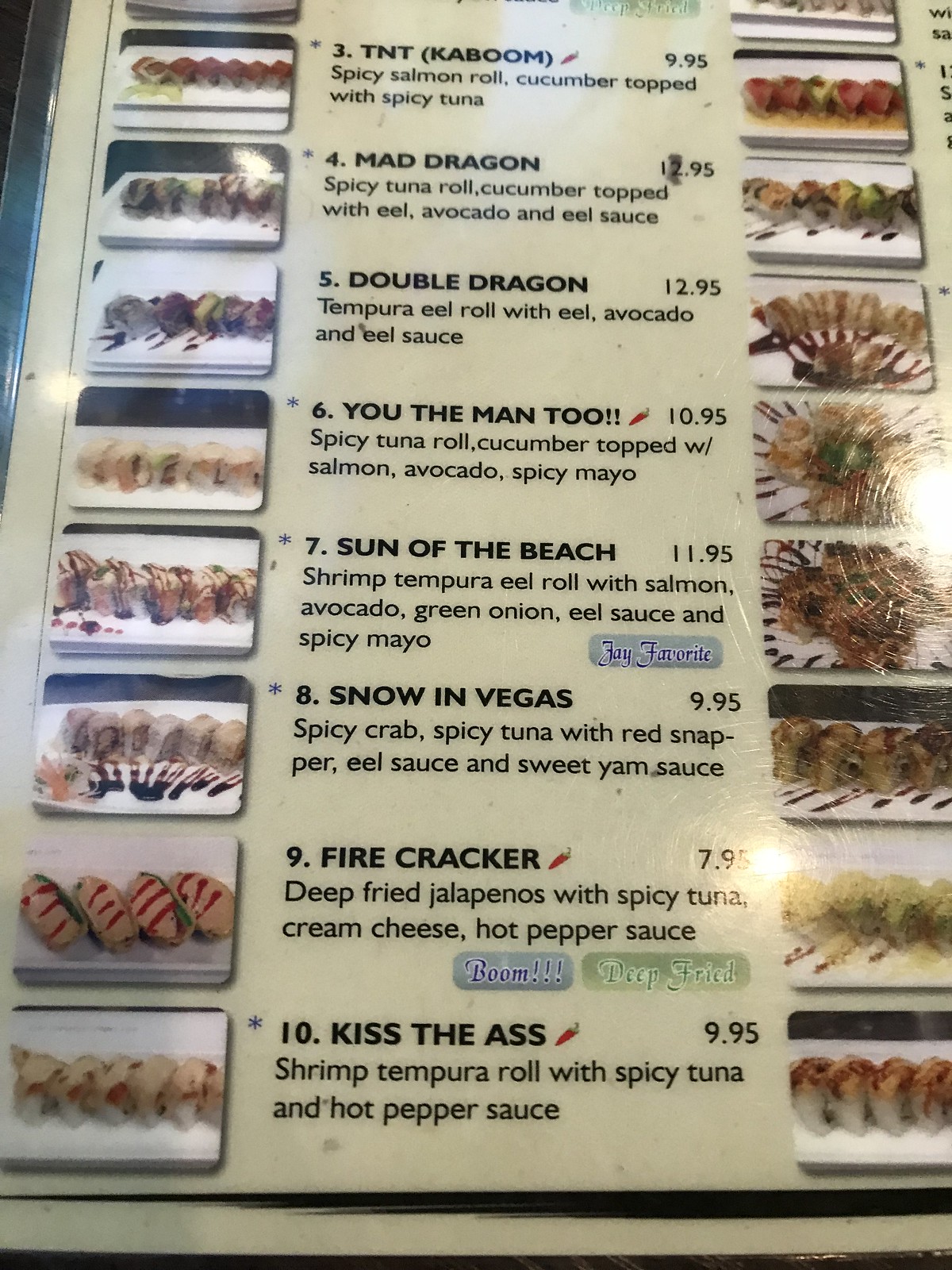The image depicts a vertically oriented menu from a Japanese restaurant, encased in a protective long rectangular plastic cover. The background of the menu is a very light, almost pastel green. The top left corner features a plastic tab, indicating the protective cover. 

At the very top of the menu, there is an item labeled "TNT Kaboom" in black text, accompanied by an image of the dish. Below it, the description reads "Spicy Salmon Roll, Cucumber Top with Spicy Tuna," and the price listed on the right side is $9.95.

Beneath the "TNT Kaboom" item, the menu continues with several more sushi options, each with the name and corresponding image of the dish on the left side:

- "Mad Dragon"
- "Double Dragon"
- "You the Man 2"
- "Son of the Beach"
- "Snow in Vegas"
- "Firecracker"
- "Kick the Ass"

Each item features a mouth-watering image of the sushi, providing a visual reference for the customers. The right side of the menu is also adorned with additional pictures of various sushi dishes, enhancing the visual appeal and helping diners make their selection.